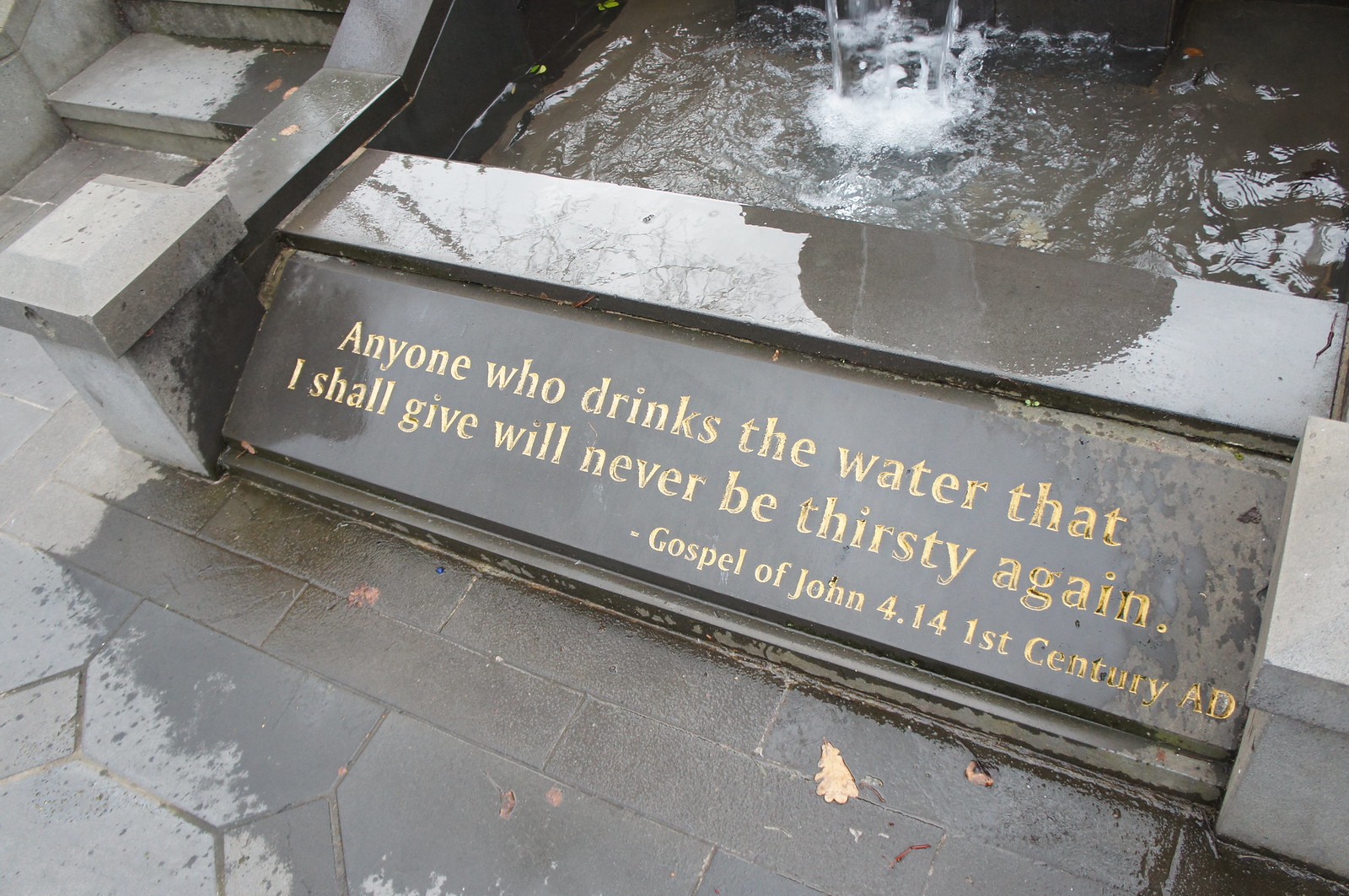In this image, we see a detailed scene of a concrete and marble water fountain, prominently featuring a gold-inscribed plaque with the biblical quote, "Anyone who drinks the water that I shall give will never be thirsty again." Below this quote, written in smaller text, is the citation: "Gospel of John 4:14, 1st century AD." The inscription is visibly wet, with water splashes covering the plaque and the surrounding area. The fountain spills water into a pool at its base, further emphasizing its active state. The ground around the fountain is paved with varied stone shapes, including rectangles, pentagons, and diamonds. In the top left corner of the image, there are tan stone steps with a handrail ascending past the fountain, suggesting this area is part of a larger, possibly ecclesiastical structure, like a church. The stone structure and intricate design details give the scene an aura of historical and religious significance.